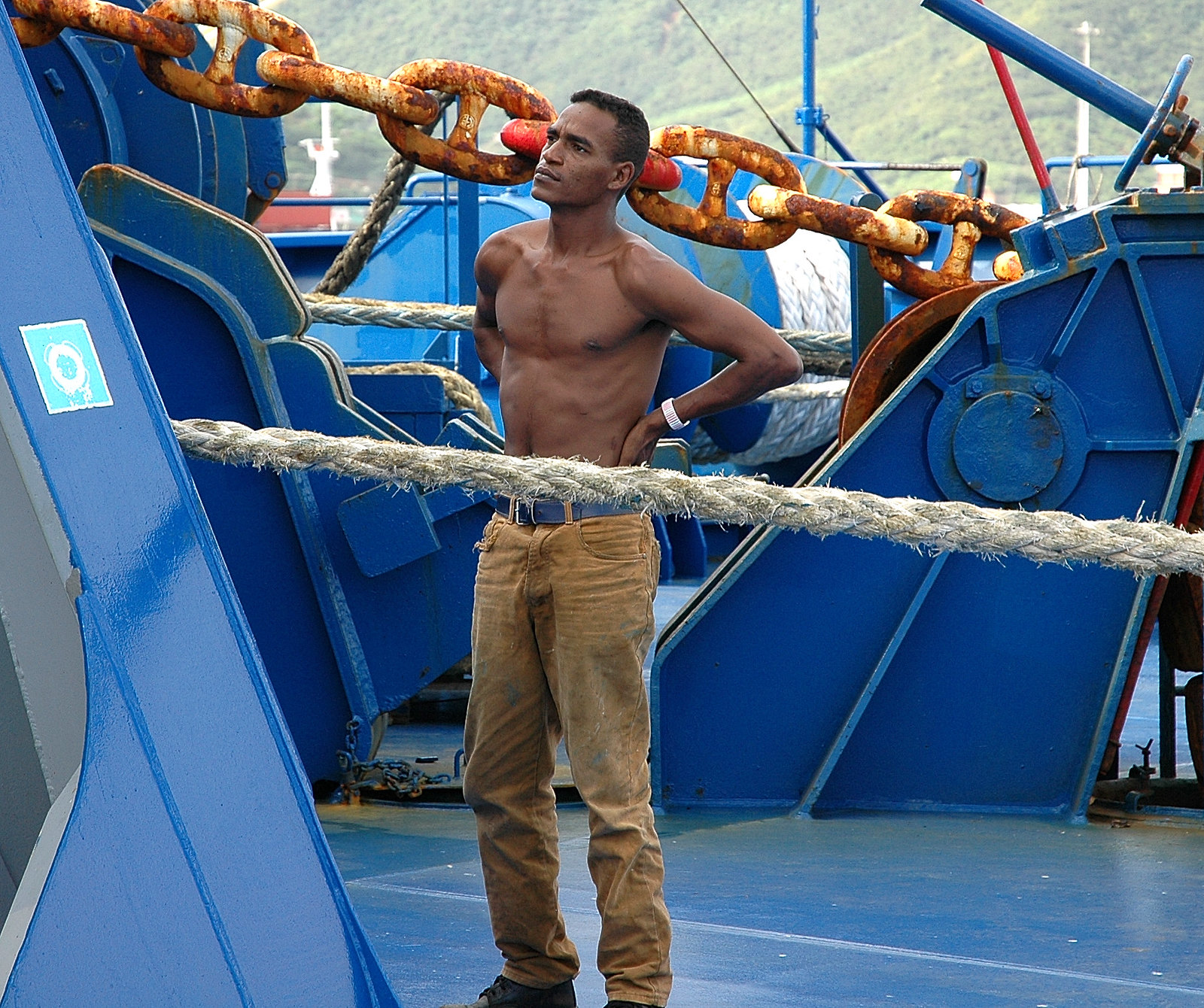The photograph captures a shirtless man of African descent standing confidently on the deck of a ship. He is dressed in brown khaki work pants secured with a black leather belt featuring a silver buckle, and black tennis shoes with coordinating black laces. A white wristwatch adorns his left wrist as he stands with his hands on his hips, looking to the left side of the image. Dominating the foreground is a thick, white-framed rope that runs from the front edge of the photo towards the man. The ship's deck, painted a vibrant blue, is also dotted with multiple winches, cranes, and chains, adding to the industrial ambience. Behind the man, a significant portion of the photograph is occupied by a large, rusted chain that once was white, stretching horizontally. In the distance, the faded background hints at lush, green hills or mountains, suggesting a picturesque contrast to the rugged maritime setting.